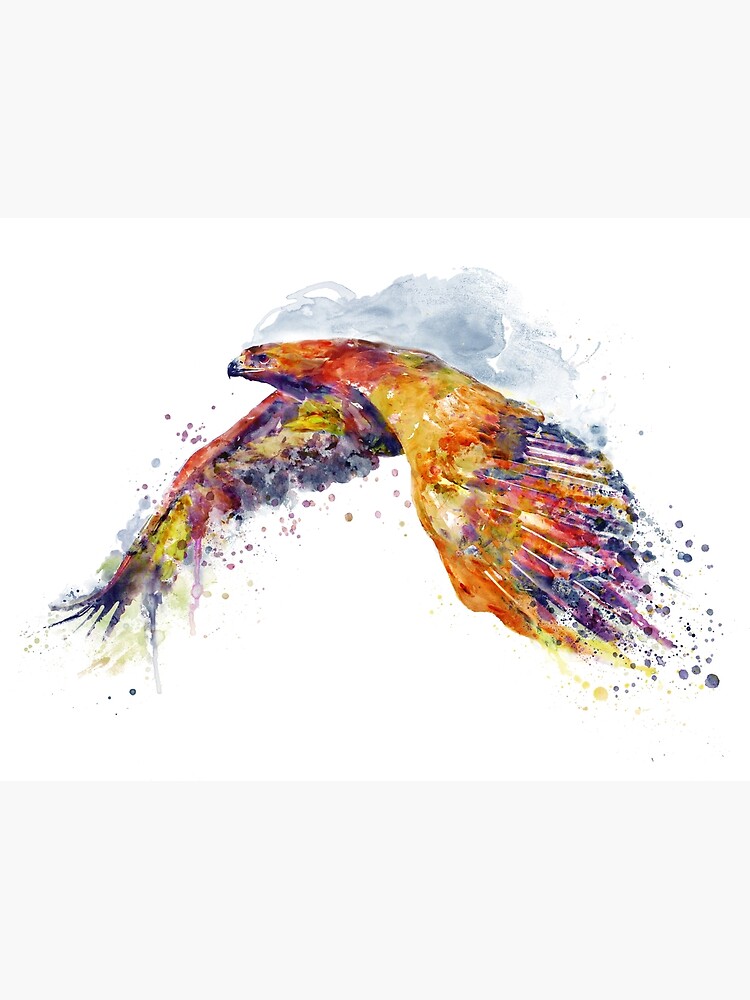This illustration, likely a watercolor painting, features a majestic bird of prey, possibly a hawk, falcon, or eagle. The bird is rendered in an array of extremely vibrant, almost psychedelic colors, including yellows, purples, reds, oranges, and blue-blacks, which is atypical and gives the piece a surreal quality. The bird's body has a striking yellow-orange hue, while its wingtips are accented with purples and grays. The bird's head is notably sharp-billed, enhancing its predatory appearance. The painting captures the bird mid-flight, with its wings flapping downward as if pushing the air beneath it. Above the bird hovers a grayish cloud formation, which might represent the speed of its flight or serve as a backdrop. The overall composition on a white background emphasizes the bird's vibrant colors and dynamic motion.